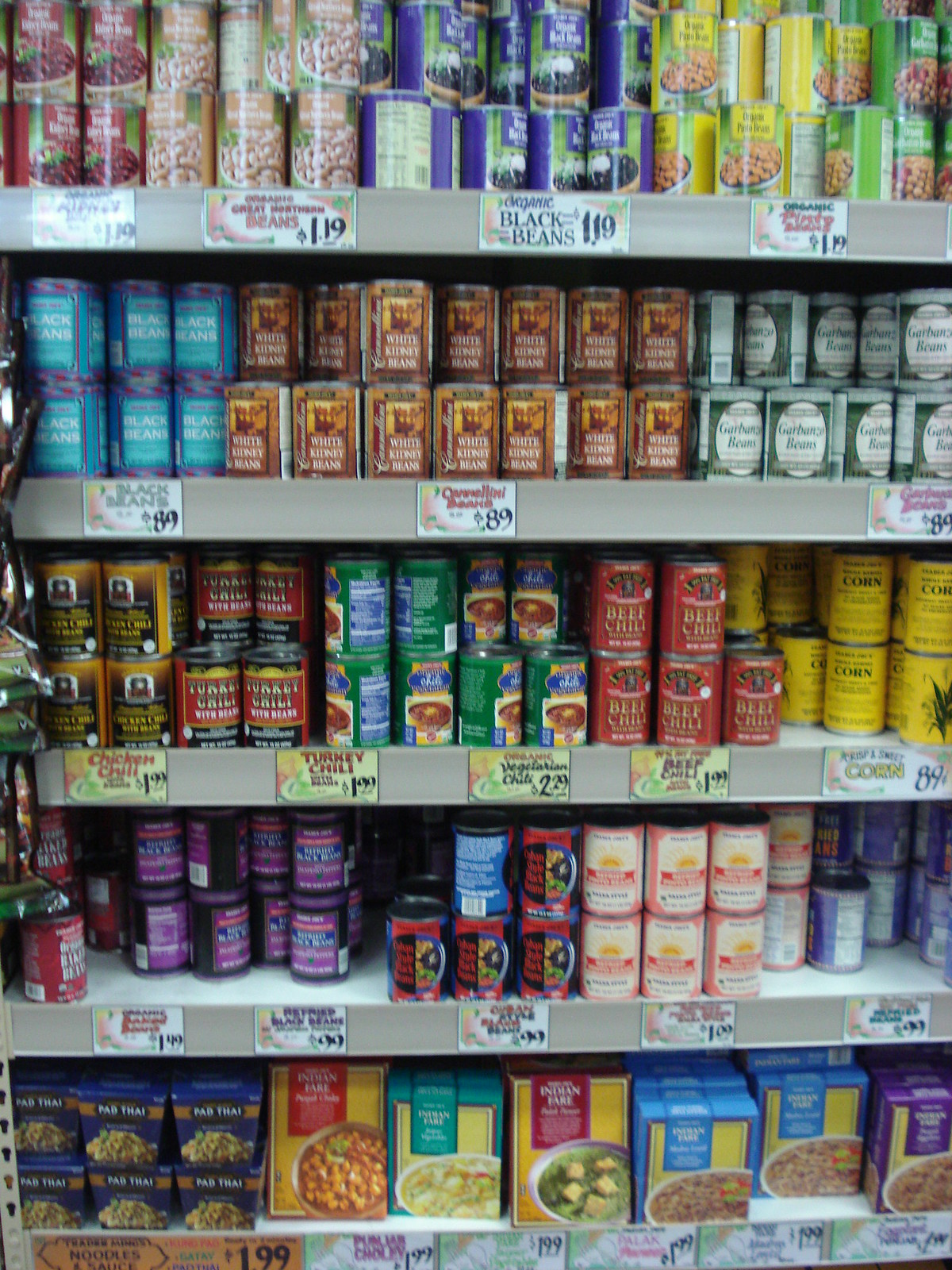The image captures an aisle in a grocery store, specifically the section dedicated to canned and dry goods. The shelves are organized with various items including organic black beans, pinto beans, turkey chili, beef chili, and canned corn. Lower shelves feature an assortment of stir-fry mixes and boxed goods labeled with international flavors, such as Thai. The products are displayed on heavy-duty metal shelves with gray trim. Prices are clearly marked, with canned items around $1.99 to $2.29. The aisle offers diverse options to cater to different culinary tastes, from traditional beans and chilis to exotic flavors and spices, indicative of a well-stocked store with a focus on both local and imported goods.